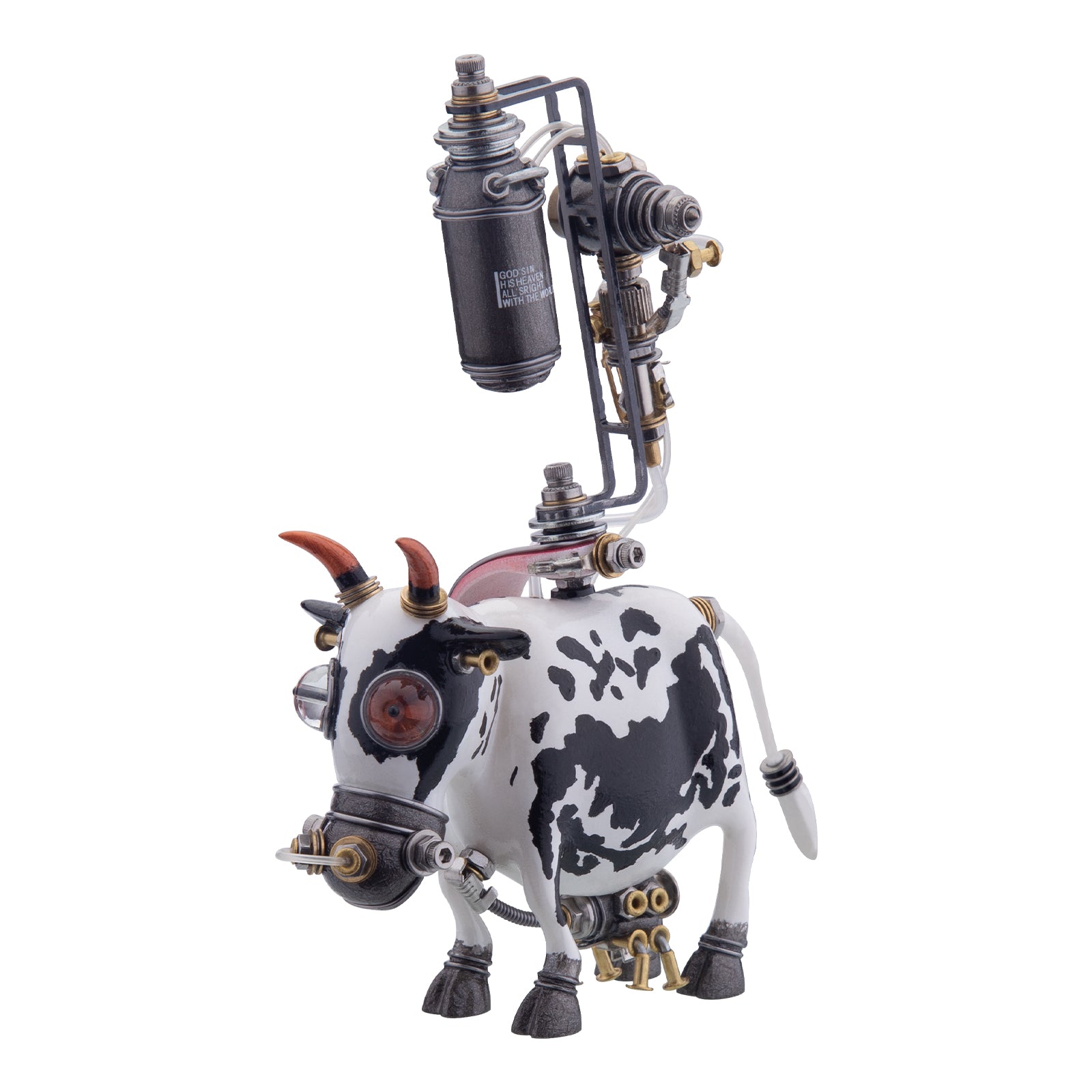The image depicts a peculiar metallic or ceramic statue of a dairy cow, primarily white with black spots, set against a plain white background. This steampunk-inspired cow features multiple mechanical elements: red and clear light bulb-like eyes, red horns adorned with tiny gold rings, and a muzzle equipped with gold bolts and a connecting tube. The robot-like figure stands facing left, with gray metal hooves and a futuristic udder replacing the usual one, complete with golden teats and an adjoining gray pump machine. Above its back is an elaborate assembly resembling an oxygen tank or jet pack, embellished with brass fittings, metal bars, and tubes. Inscribed on the black tank are the words, "God's in his heaven, all's right with the world." The statue is roughly five inches high and three inches wide, with meticulously crafted details that blend whimsy and technology seamlessly.